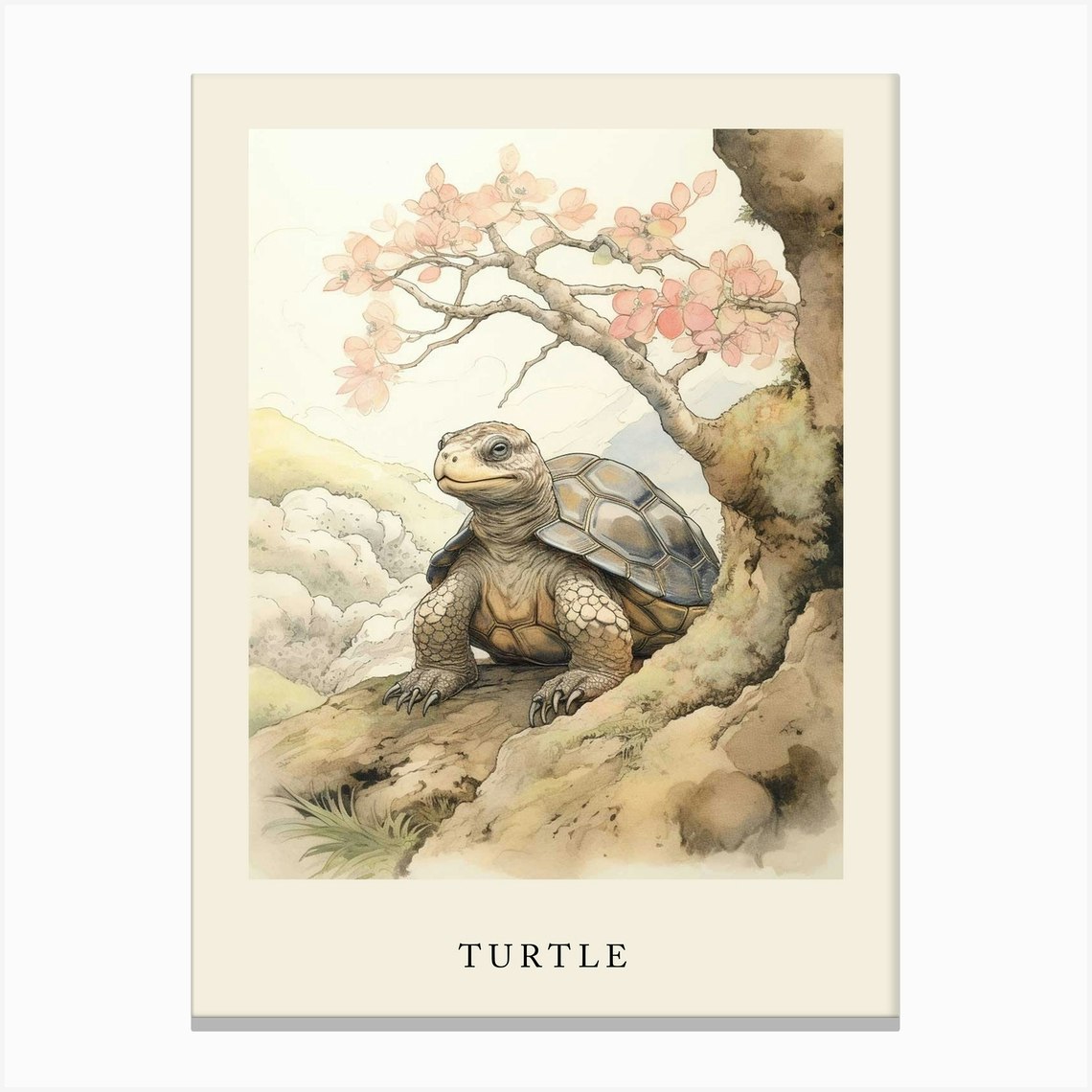This image features a vertical rectangle composition with a light gray outline and a white border that is slim at the top and bottom but wider on the left and right. Nested inside this is another vertical rectangle edged in gray, with a thin pink border on the top, left, and right, while a thicker pink border defines the bottom. 

Within this pink-bordered frame, an exquisitely detailed illustrated scene unfolds—resembling a delicately crafted postcard, possibly rendered in watercolor and pencil or pen. At the heart of the image is a beige and sandy-colored turtle, its shell a contrasting gray. The turtle faces slightly to the left, displaying front legs that extend outward, each paw armed with sharp talons. 

To the right of the turtle, a rocky ledge juts into the scene. From this ledge, a gnarled tree with pink blossoms reaches upward to the left, its branches creating a canopy above the turtle. To the left, in the distance, a hillside dotted with rocks and a few bushes extends the scene.

Foreground details include sprigs of grass interspersed among the roots of the tree, all set against a landscape of rocky terrain. The sky is a simple, clean white backdrop, allowing the earthy tones and delicate pinks of the illustration to stand out. Anchoring the image, at the bottom, the word "TURTLE" is prominently displayed in all capital black serif letters within the thick pink border.